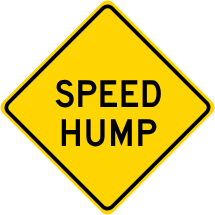This image depicts a diamond-shaped traffic sign set against a white background, with no pole or mounting structure. The sign features a bright yellow field with a subtle yellow outer trim, bordered on the inside by a bold black outline. At the center, in large, capitalized black sans-serif font, the sign reads "SPEED" on the top line and "HUMP" on the bottom line, perfectly centered both vertically and horizontally. The text is clear but might have slightly blurry edges. The sign appears perfectly symmetrical and clean, with rounded corners, and serves as a caution to alert drivers of an upcoming speed hump.